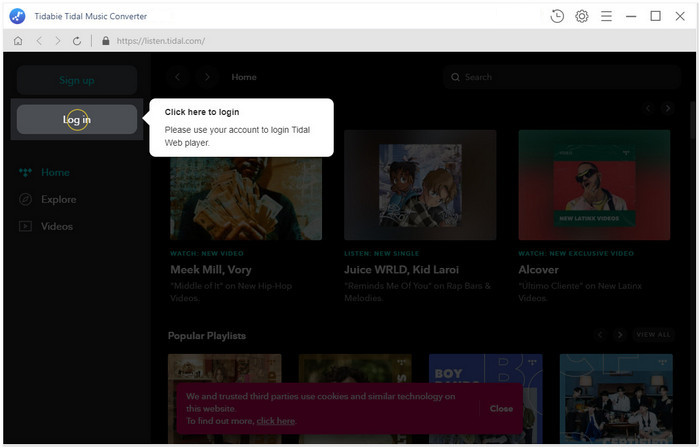The image depicts a user interface of the Tidabi Title Music Converter software, designed to convert music from Tidal to alternative formats. The software interface sports a dark theme with most elements appearing in varying shades of gray. Notable within the interface is a login button located on the right side of the screen. When hovered over, a tooltip appears with the message: "Click here to log in. Please use your account to log in to Tidal web player." This suggests that users must first log in to their Tidal account to begin the conversion process.

The left sidebar of the interface includes navigational options labeled "Home," "Explorer," and "Videos." Under the "Home" section, album covers are displayed, featuring artists such as Meek Mill and Juice WRLD. Although the full list is not entirely legible, popular playlists are presented towards the bottom of the panel. The URL provided, "listen.tidal.com," indicates a direct link to the Tidal web player, an essential step for users to log in and access their music for conversion.

Overall, the image effectively showcases the Tidabi Title Music Converter as a tool designed to simplify the process of converting Tidal music to different formats, likely to manage file sizes or enhance compatibility with various devices.